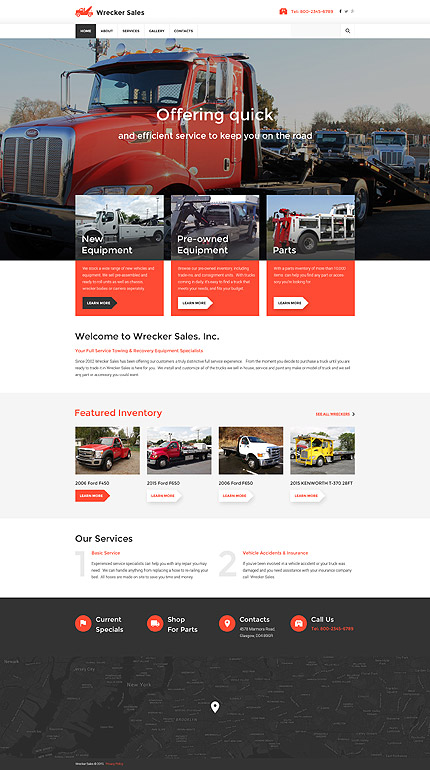The full-page depiction appears to be a mobile website layout presented as one continuous image, eliminating the need for scrolling. 

At the top left, the "Wrecker Sales" logo prominently features a red silhouette of a wrecker vehicle adjacent to the company name. To the right of the logo, a phone number is displayed alongside three tiny social media icons.

Directly below this section, towards the center left, five categories are listed in small black text, with the first category currently highlighted. 

Dominating the page is a large image of a semi-truck equipped with a wrecker bed. Superimposed at the center of this image are the words "Offering Quick," followed by smaller white text beneath them.

At the bottom center of this section, three smaller thumbnail images are aligned horizontally, each with a red box and white descriptive text below them. An arrow adjacent to these thumbnails invites viewers to "click here to learn more."

Further down, the text "Welcome to Wrecker Sales, Inc." is centered prominently on the page, followed by a short description introducing the company.

In the middle of the page, a large gray box with the heading "Featured Inventory" in orange houses four thumbnails of different vehicles. Each thumbnail has a price displayed underneath, and arrows encouraging further clicks for more information.

The bottom section of the page is dedicated to the "Our Services" category. On the left, a large gray number "1" is paired with an accompanying paragraph, and to the right, a large gray number "2" is similarly accompanied by a descriptive paragraph.